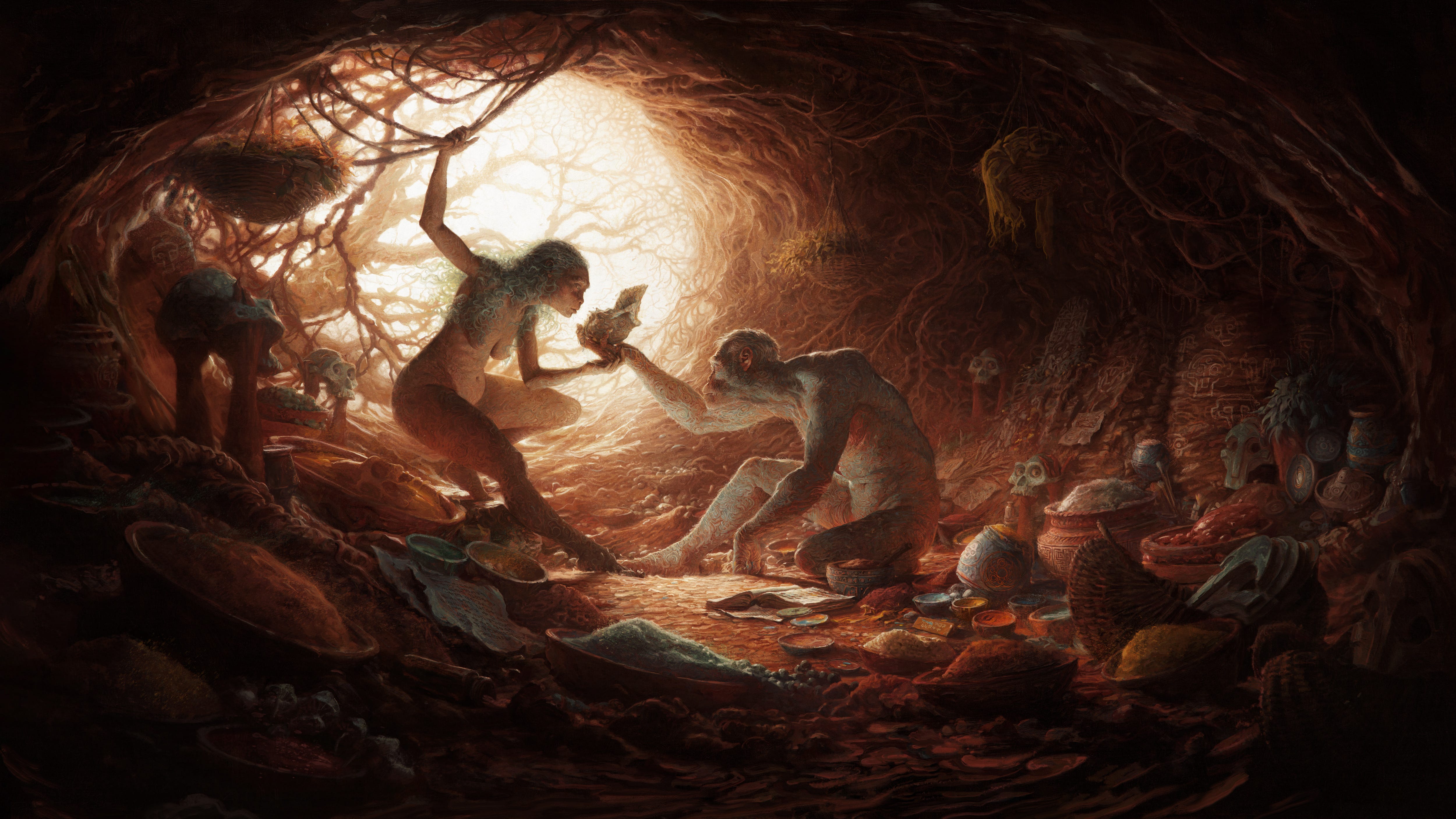In the artist's detailed drawing of an ancient cave interior, we see a nude female figure distinguished by very archaic facial features, holding onto a vine hanging from the cave ceiling. Her right leg is extended forward, resembling the poised stance of a dancer. To her right is a male figure, characterized by similarly ancient facial structures and a slight back hump, sitting with his right leg stretched out and his left arm resting on the ground. He is handing an object to the female, and both appear deeply engaged with each other. 

The cave floor is rocky and strewn with various items, including crude implements, vases, jars, baskets filled with tomatoes and rice, and bowls. Scattered across the cave walls are skeletal skulls and faint markings, enhancing the primitive atmosphere. The cave’s interior transitions from brown hues at the sides to black at the top, while sunlight shines through the entrance, illuminating a tree silhouetted against the light. Vines and branches overgrow the cave’s entrance, adding to the ancient, mystical ambiance.